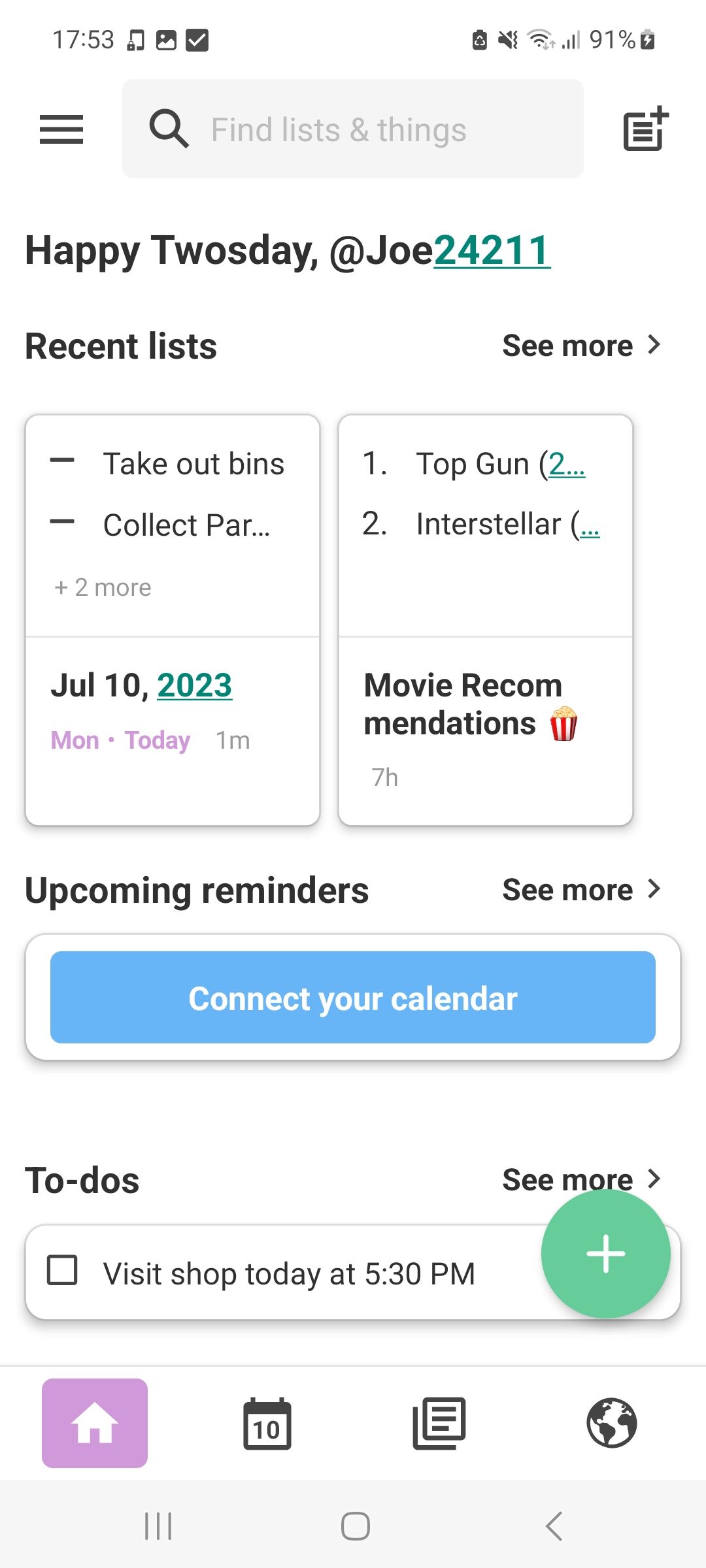This screenshot, taken from a phone at 5:53 PM with a 91% battery, features a user interface with a hamburger menu icon on the left and a search bar with a magnifying glass labeled "Find list and things." Below this, it greets the user with "Happy Tuesday @Joe 24211."

The screen displays multiple sections:

1. **Recent List**: 
   - A section titled "Recent List" with an option to "See more." 
   - The left box highlights tasks such as "Take out bins and collect P.A.R." along with two more tasks, all scheduled for "July 10th, 2023, Monday, today, one minute."
   - The right box shows movie recommendations with a popcorn icon, listing "1. Top Gun" and "2. Interstellar."

2. **Upcoming Reminders**:
   - This section encourages the user to "See more" and "Connect your calendar" within a blue box.

3. **To-dos**:
   - The To-dos section with an option to "See more" and a plus sign to add new tasks.
   - A listed task for today at 5:30 PM to "Visit shop," marked with an unchecked checkbox.